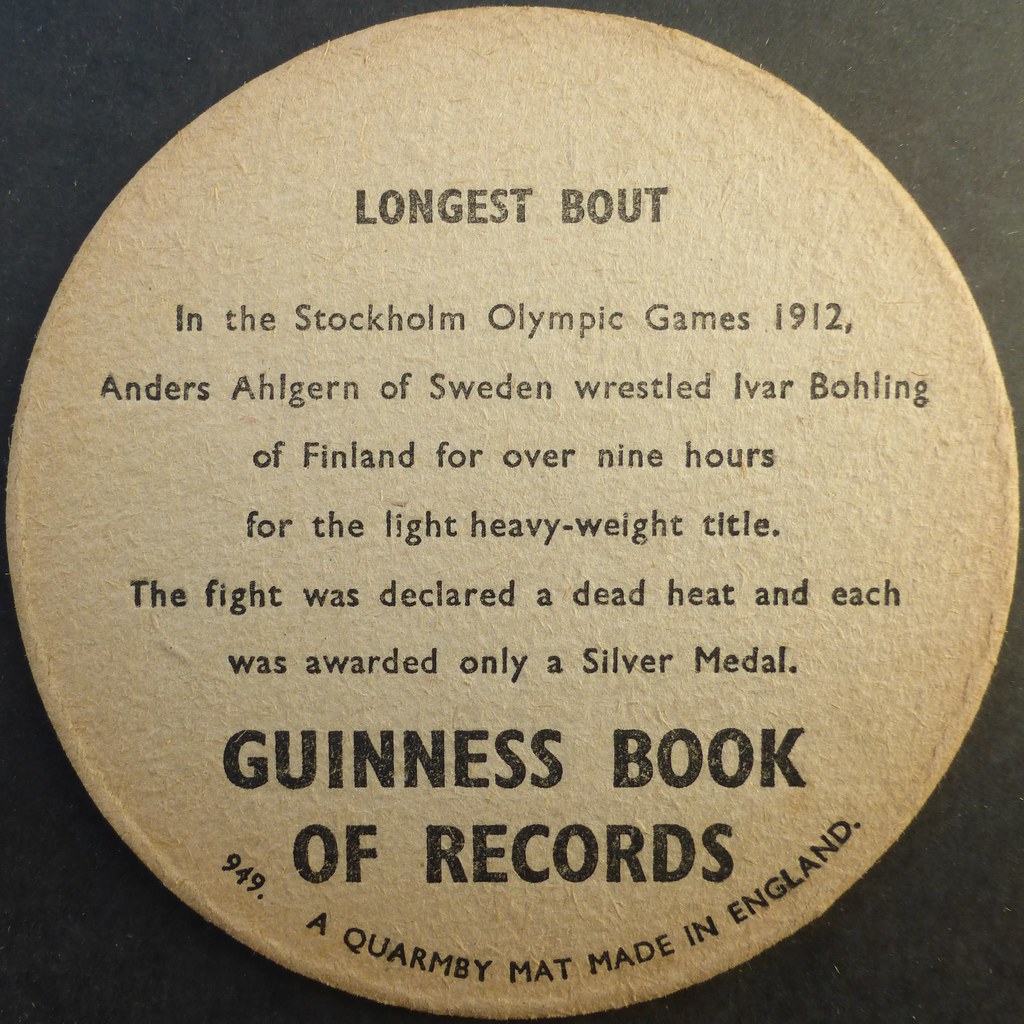This image features a closely zoomed-in view of a round, tan coaster, possibly made of cardboard, positioned against a black table. Dominating the coaster's surface, the title "Longest Bout" is boldly printed at the top in spaced out, easy-to-read black letters. Beneath the title, in smaller but clear black print, a detailed account from the Guinness Book of World Records reads: "In the Stockholm Olympic Games 1912, Anders Ahlgren of Sweden wrestled Ivar Böhling of Finland for over nine hours for the light heavyweight title. The fight was declared a dead heat and each was awarded only a silver medal." At the bottom, giving credit, the text states "Guinness Book of Records" again in larger, bold letters, followed by "949.8 Quornby mat, made in England." The coaster, devoid of any images or additional graphics, emphasizes a British origin with its textual content and historical reference, maintaining a vintage and informative aesthetic.